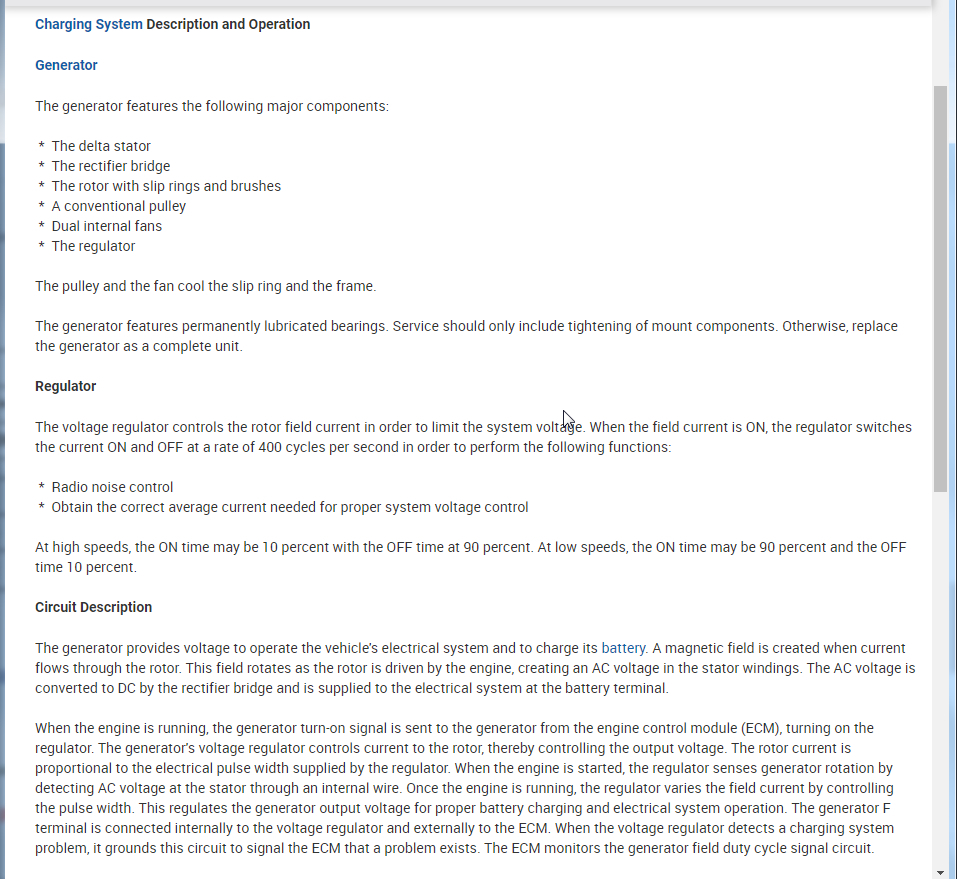**Detailed Caption: Charging System Description and Operation**

The image displays an instruction page detailing the charging system's description and operation for a generator. The background of the page is white. In the upper left corner, there is prominent blue text stating "Charging System," followed by black text saying "Description and Operation." Further below, blue text introduces the term "Generator" and is followed by black text listing its major components:

1. The Delta Stator
2. The Rectifier Bridge
3. The Rotor with Slip Rings and Brushes
4. A Conventional Pulley
5. Dual Internal Fans
6. The Regulator

It is noted that the pulley and the fan are responsible for cooling both the slip ring and the frame. Additionally, the generator features permanently lubricated bearings, and service should generally be limited to tightening mounting components; otherwise, replacing the generator as a complete unit is recommended.

Below this section, there is a heading for "Regulator," followed by a description detailing the Voltage Regulator, which controls the rotor field current to maintain system voltage. The regulator's functionality involves switching the field current on and off at a rate of 400 cycles per second to control radio noise and achieve the correct average current for proper system voltage control. The duty cycle of this switching varies with speed: at high speeds, the "on" time may be 10% and the "off" time 90%, whereas at low speeds, the "on" time may be 90% and the "off" time 10%.

The caption then gives an overview of the Circuit Description, stating that the generator provides voltage to operate the vehicle's electrical system and charge its battery. The generation of a magnetic field in the rotor, which is driven by the engine, creates an AC voltage in the stator windings. This AC voltage is then converted to DC by the rectifier bridge and supplied to the battery terminal. When the engine runs, the generator receives a turn-on signal from the engine control module (ECM), activating the regulator. The Voltage Regulator manages the current to the rotor, thus controlling the output voltage. The rotor current is proportionate to the electrical pulse dictated by the regulator.

Upon starting the engine, the regulator senses generator rotation by detecting AC voltage at the stator through an internal wire. After detecting rotation, the regulator adjusts the field pulse width to regulate the output voltage for efficient battery charging and electrical system operation.

Finally, the image details that the generator F terminal connects internally to the voltage regulator and externally to the ECM. In cases where the voltage regulator identifies a charging system issue, it grounds the circuit to alert the ECM. The ECM, in turn, monitors the generator field duty cycle signal circuit.